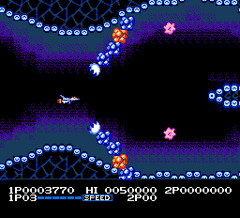The image is a detailed screenshot from an early Atari-era video game. It depicts an underwater scene with small, white bubbles at the top and bottom edges of the screen, accentuating the aquatic environment. The center of the screen is predominantly black, flanked by dark gray areas that enhance the sense of depth. In the very center-left, there's a small spaceship flying through what appears to be a rocky, fenced area, potentially representing underwater rocks or bubble barriers. On the right side of the screen, the spaceship seems poised to navigate around another bubble-like structure.

At the bottom of the screen, the user interface shows the in-game score in a classic Atari-style font, reading "1P0003770", suggesting it is Player 1’s score. Additional HUD elements include a black rectangle with white text displaying "1P03". Above that, in a blue rectangle, the spaceship's speed is indicated. The high score "HI 0050000" is also prominently shown, signifying a target for the player. More detailed elements like "2P00" and "2P00000000" reference Player 2’s scores or potential stats, although specifics aren't entirely clear from the image.

The image also features a narrow tunnel opening into a larger space, emphasizing a constrained flight path widening into a more open area. Two creatures are illustrated, one on the ground and one hanging from above, both extending towards the spaceship. There are also small, star-like bursts at the top and bottom of the screen. A subtle "V" shape of light emanates from the right side, adding to the game's vintage graphics flair.